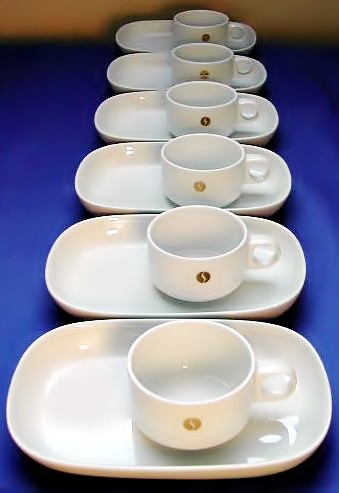The photograph depicts six identical white ceramic teacup and rectangular plate sets arranged neatly on a navy blue tablecloth. Each shallow cup, which could also serve as a coffee mug, features either a yellowish or a brownish logo or decal on the front, alternating between the two colors. The logos appear to be small circular emblems with a curved line in the center. The rectangular plates, also white ceramic and shiny, are placed with the cups positioned more towards the right side. The setup is likely for a meal, possibly at a restaurant, and the entire arrangement rests on a vibrant blue tablecloth beneath a light tan wall.